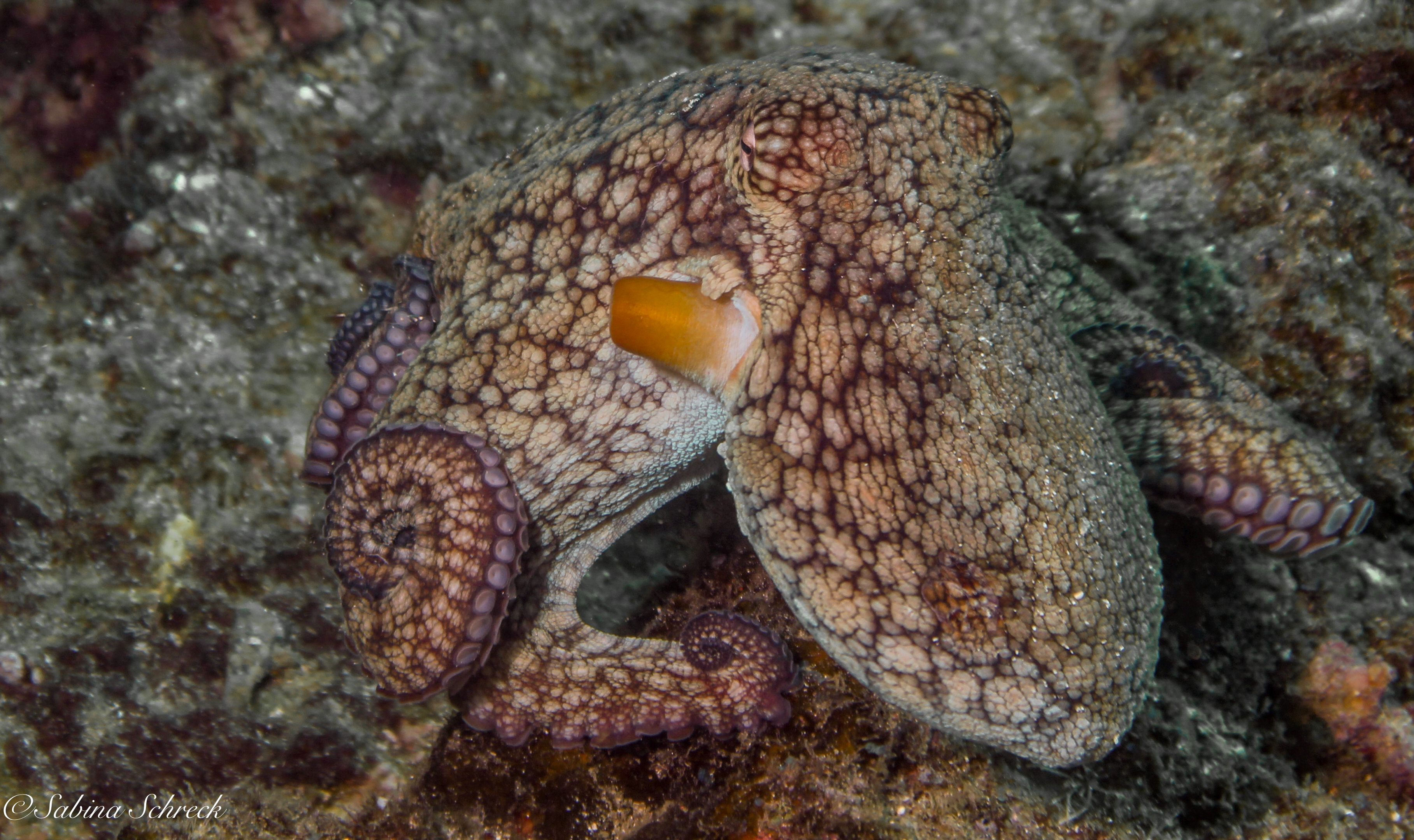This underwater photograph showcases a masterfully camouflaged octopus on a variegated crystalline, rocky surface that transitions in color from golden hues to grays and browns. The octopus has expertly blended into its surroundings, adopting the same gold, gray, and brown tones. In the foreground, the tentacled legs, visible towards the lower left, display suckers that are subtly apparent. A significant focal point in the center of the image is an orange-yellow tube, situated on the side of the octopus's face, which intriguingly resembles a duck bill. The texture of the octopus's skin and its camouflage make it challenging to spot, with even its circular eyes, appearing almost closed, adding to the disguise. The rocky surface beneath the octopus accentuates the intricate details of the creature's mimicry. At the bottom left of this professional capture is the photographer's name, Sabina Schreck.